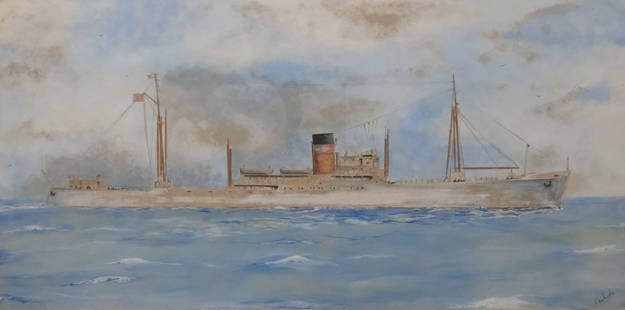The painting depicts a large, substantial ship, likely a 19th-century steamboat, occupying nearly the entire horizon from left to right. The vessel, predominantly white with gray sections, is characterized by a prominent orange smokestack with a black top situated at its center. Two masts tower at either end, connected by a series of wires. The ship sails on gently wavy, deep blue water, evoking a tranquil scene. The sky above is dense with dark, heavy clouds interwoven with patches of blue and pink, suggesting an impending storm. The artist has signed their work in the bottom right corner of the painting.